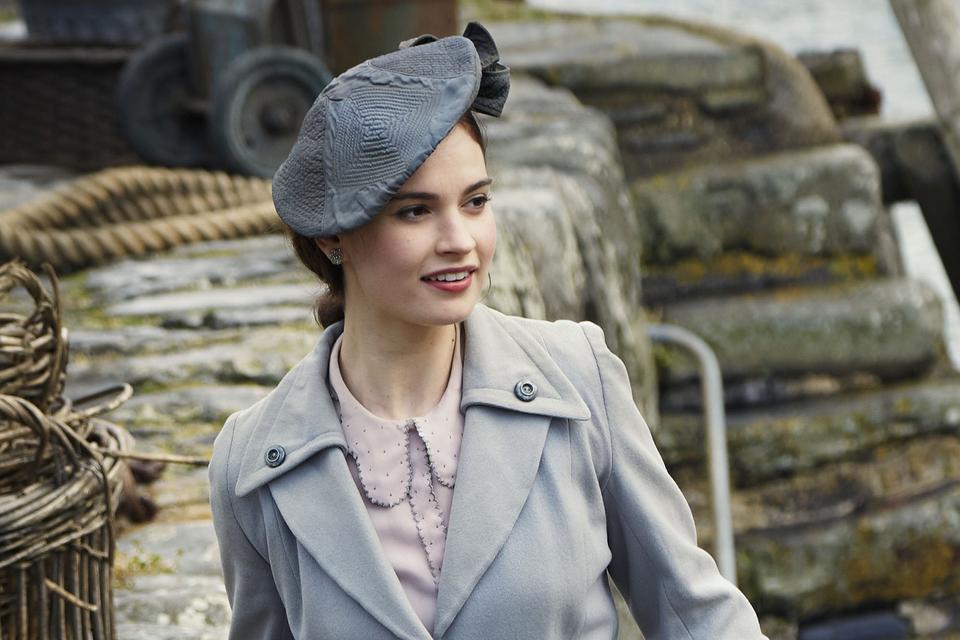This daytime outdoor photograph features an elegantly dressed woman, possibly an actress, positioned centrally in the image from her midsection up. She has her face turned to the right, smiling with visible red lips and looking as though she sees someone. She is dressed in a stylish gray overcoat with a large collar, which covers a collared undershirt in a light lilac or off-white color. Atop her head, she wears a gray knitted beret adorned with a bow or ribbon. A single earring is visible on her exposed ear. The background showcases a rustic setting, including a moss-covered stone wall with light tan ropes and wicker baskets arranged to her left, as well as what seems to be stone stairs on her right. The scene exudes a sense of classic charm and timeless elegance.